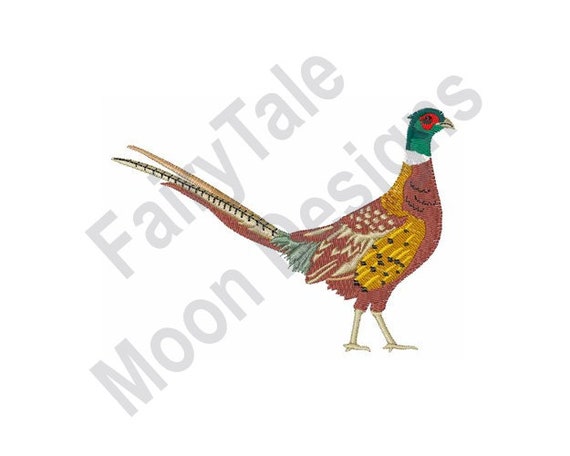The image appears to be a digital artwork or possibly an embroidery of a ring-neck pheasant, which might also be used as a stitched patch for garments or accessories. The bird is intricately detailed, featuring a distinct green head with red markings around the eyes and a white ring around its neck. Its body exhibits a rich brown color with gold hues on the wings and back, complemented by light cream spots on the wings. The tail is elongated with feathers in shades of whitish, beige, and brown, while the rump displays a unique teal coloration. The legs are a light beige. Notably, the background includes a transparent watermark reading "Fairytale Moon Designs," indicating its origin and serving as a copyright measure to prevent unauthorized use.